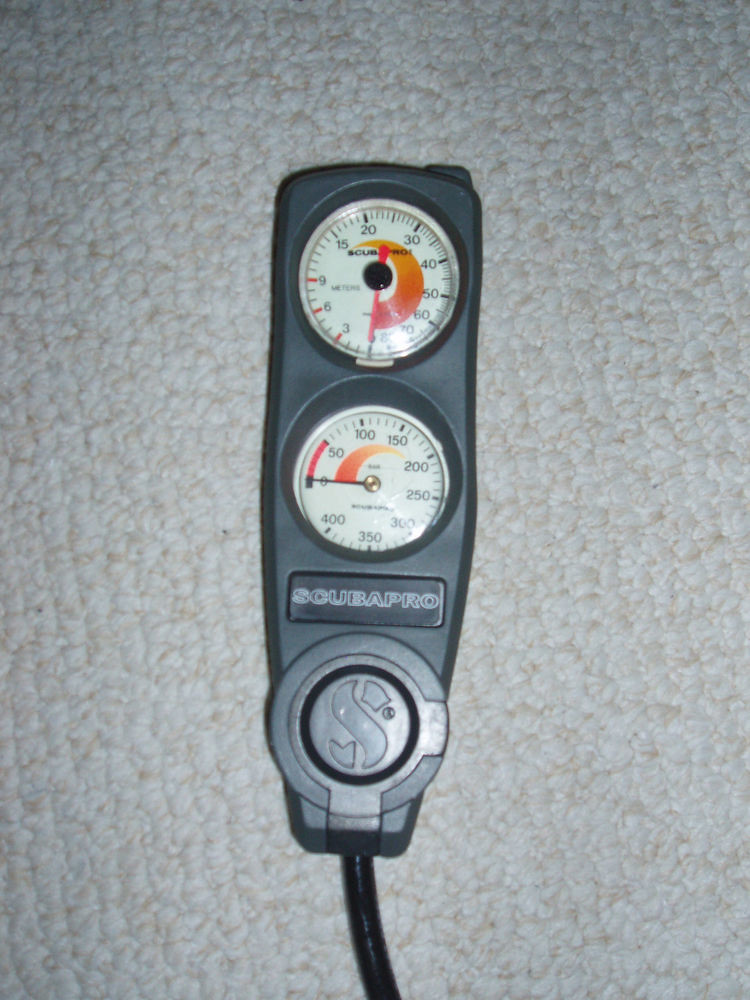This image features a poorly lit photograph with a white Berber carpet serving as the backdrop. Dominating the center of the image is a black plastic gauge, which is rectangular in shape but tapers toward the bottom. Emerging from the tapered end is a black wire extending towards the bottom-right corner of the frame. 

The gauge itself has a dual-dial design. At the top of the black rectangular structure, there is a gray plastic frame encasing a white clock-face dial, numbered from 1 to 20 in a vertical arrangement, with 1 at the bottom and 20 at the top. A small red arrow, presumably movable, is used to indicate measurements. The word "scuba" is clearly printed in the center of this dial.

Below this is a second white dial, also resembling a clock face, but this one is marked from 0 to 400. The black arrow indicates the measurement on this scale. The lower section of the gauge prominently features the brand name "Scubapro" written in white font. This appears to be a specialized device used in scuba diving.